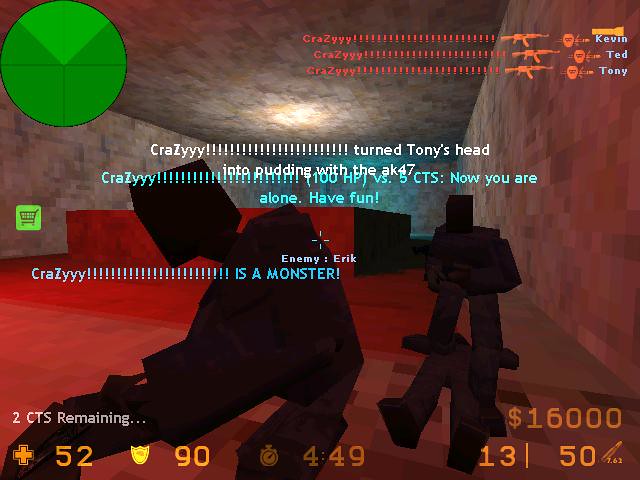This image is a detailed, color screenshot from an animated video game scene. The graphics are notably blocky and primitive, with a 3D effect. The scene takes place in a room with gray walls and ceiling, a red floor, and light tan brown walls in some parts, illuminated by blue and red lights. Black, humanoid figures featuring square and rectangular body parts, resembling dark silhouettes, populate the foreground.

In the top left corner of the screen is a small green segmented circle. Scattered text across the image includes red writing next to orange rifles, with names like Kevin, Ted, and Tony written in blue to the right of these rifles. The word "crazy" is prominently displayed multiple times with vibrant exclamation points. Additionally, the phrases "Turn Tony's head into pudding with the AK-47" and "Crazy 100 HP versus 5 CTS. Now you are alone. Have fun. Enemy: Eric" are written in white and blue text across the center.

A small green box with a gray shopping cart icon is also visible on the left side. At the bottom of the image, white text and abundant orange text detail various game statistics, including numbers indicating health, ammo, remaining time (4 minutes 49 seconds), money ($16,000), and other numerical information (52, 90, 13, 50).